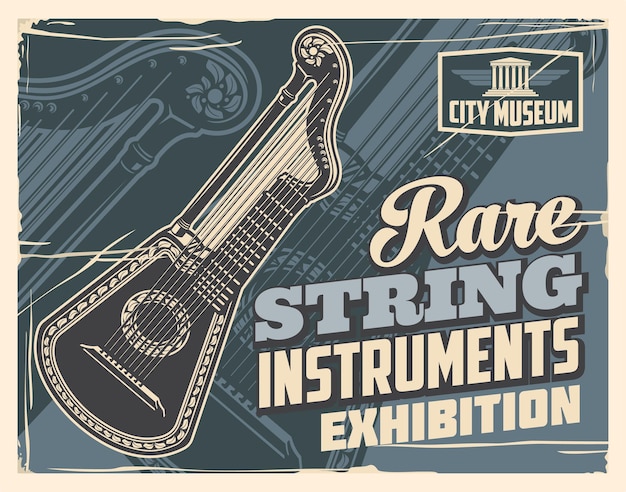This promotional poster for the City Museum's "Rare String Instruments Exhibition" features a distinctive musical illustration. At the top right, the City Museum logo, a classic Greek portico design, sets a refined tone. Below the logo, the exhibition title is presented in various eye-catching fonts: "Rare" in white italics, "String" in blue bold, "Instruments" in white with a black background, and "Exhibition" in all white text. Central to the poster is a detailed black-and-white illustration of a unique stringed instrument, resembling a hybrid between a guitar and a harp, possibly an eight-stringed variant. Surrounding it, enlarged blue-and-white details highlight the instrument's intricate design. This evocative imagery invites visitors to explore a collection of diverse and rare stringed instruments at the City Museum.